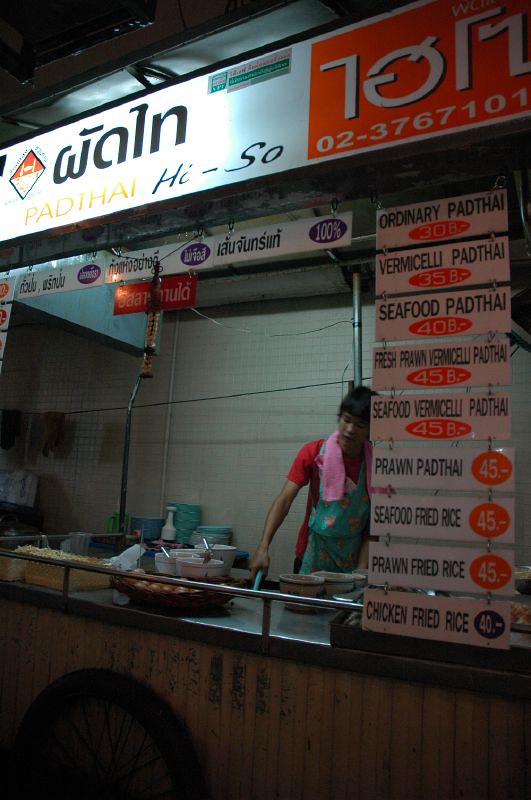The photograph depicts an outdoor food cart specializing in Thai cuisine, likely part of a bustling street food scene. A prominently lit sign at the top reads "Pad Thai," suggesting this is the main offering. The cart features a detailed menu with various Pad Thai options, including Ordinary Pad Thai, Vermicelli Pad Thai, Seafood Pad Thai, Fresh Prawn Pad Thai, Seafood Vermicelli Pad Thai, as well as different types of fried rice such as Seafood Fried Rice, Prawn Fried Rice, and Chicken Fried Rice. Prices range from 30B to 45B. A person with short black hair, wearing a red shirt under a well-worn apron, appears to be working energetically behind a steel counter. They are possibly hitting or preparing something, surrounded by numerous bowls, presumably getting ready to serve the next customer. The scene captures the lively, authentic atmosphere of a street food vendor.